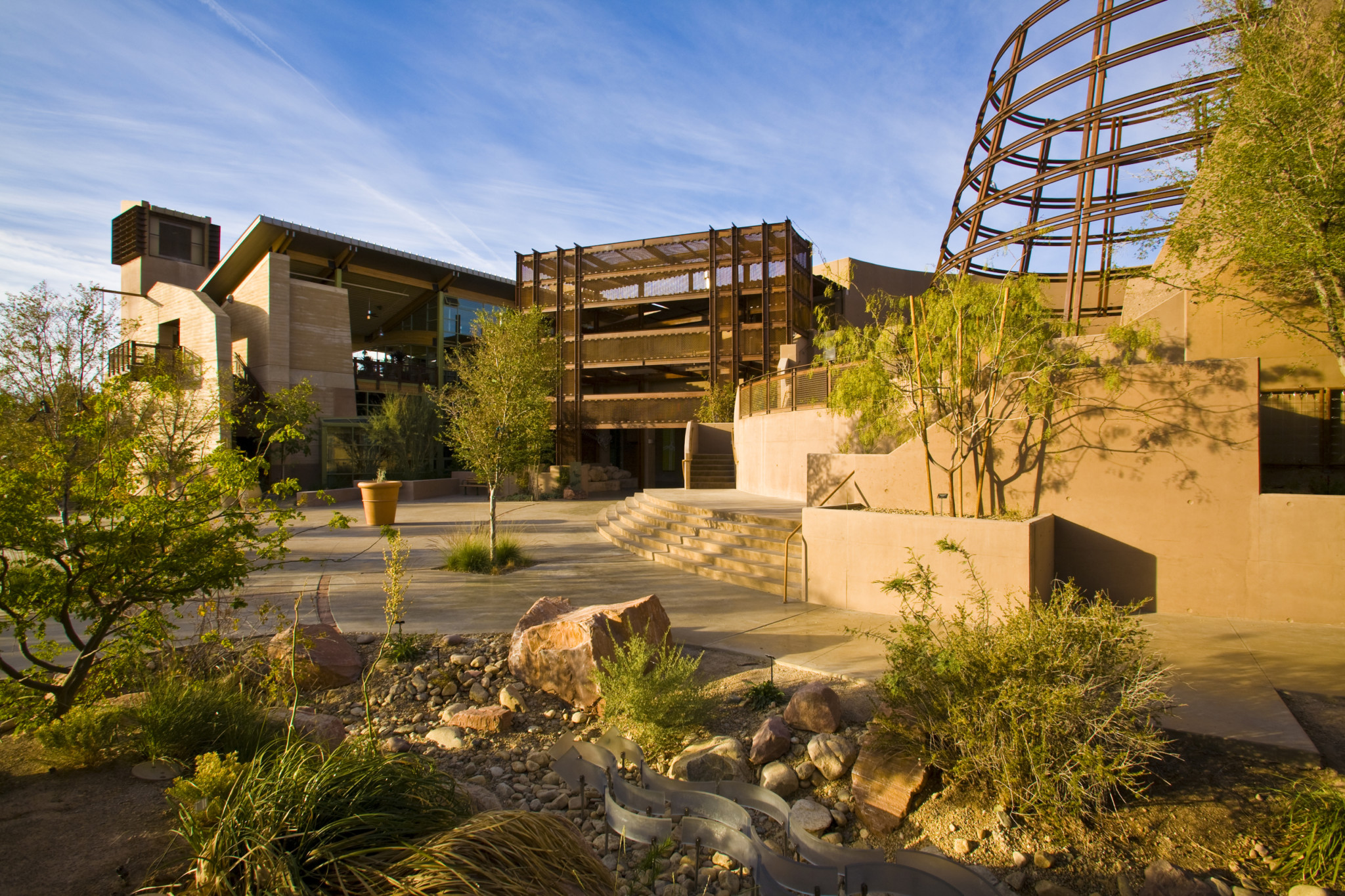Against the backdrop of a vivid blue sky adorned with white clouds, the image captures a striking modern building set in an arid desert location. Dominating the upper left-hand corner to the center of the picture, the multi-story structure features a distinctive one-pitch slanted roof and is connected to a prominent tower on the left. The foreground of the image reveals a meticulously designed garden, featuring sparse-leaved trees, scattered rocks, and patches of dirt, reflecting the arid environment. Cement walkways thread through this garden, leading to various parts of the building. The building itself appears to comprise multiple sections: the left side sports a steel circular frame with platforms and stairs, giving an industrial vibe reminiscent of a parking structure. The right side transitions into a more conventional architectural form, resembling a two or three-story residential or business facility. The thoughtful blend of modern design and natural elements creates a harmonious yet striking scene.